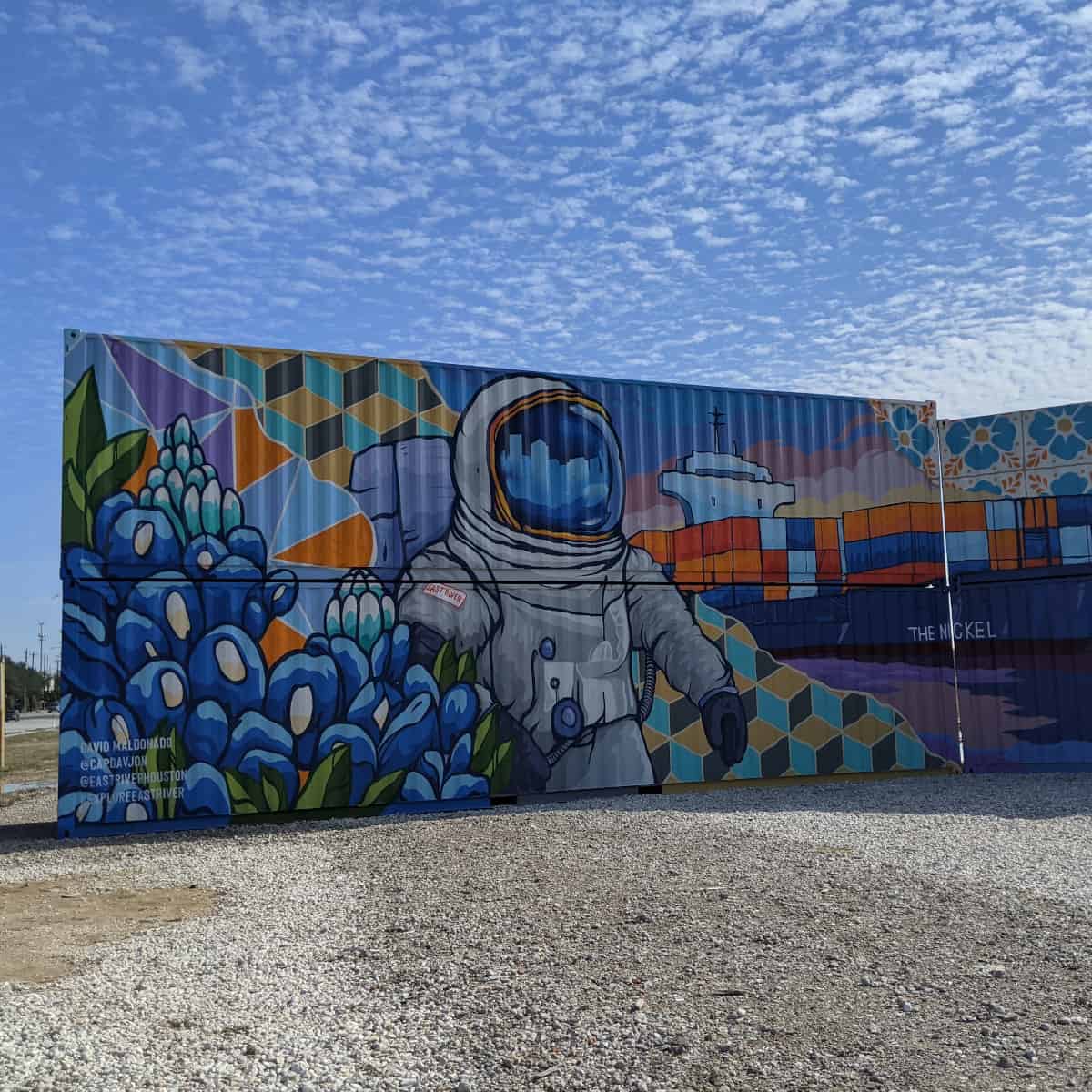The photograph showcases the renowned East River mural in Houston, Texas, beneath a patchwork of cloudy skies. This vibrant artwork is painted on the side of two stacked railroad boxcars, which are types of transport containers commonly moved by both rail and road. The mural prominently features an astronaut adorned in blue and gray, floating with black gloves against a checkerboard and cubic backdrop, with flowers and other artistic elements sprinkled across the scene. Over the astronaut's shoulder, there is a depiction of a container ship. In the foreground, gravel stretches out, while the background reveals a dirt road and power poles. The entire setup is isolated, with no visible cars or people, emphasizing the mural's solitary grandeur near what appears to be a dirt road. The mural also includes the artist's copyright, though the text is hard to discern.